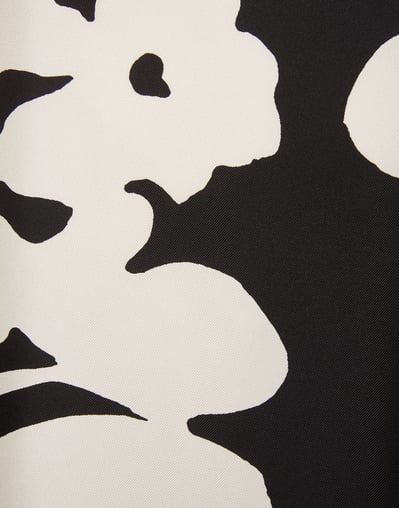The image presents an up-close, abstract depiction of a textured fabric, possibly resembling a dress or skirt, characterized by a high-contrast black and white pattern. The beige base of the fabric is markedly interrupted by a series of distinctive black marks and designs. Notably, on the top left corner, a black mark protrudes, while a larger black shape extends diagonally from the bottom right to the upper left, dominating much of the background. This dominant black area features a white untouched spot on its right side. The left side of the image primarily remains white, dotted with smaller black blotches and irregular lines which invoke the impression of florals or imaginative creatures like birds or deer. The intricate, intertwined designs invite various interpretations, suggesting a dynamic, ever-changing scene.